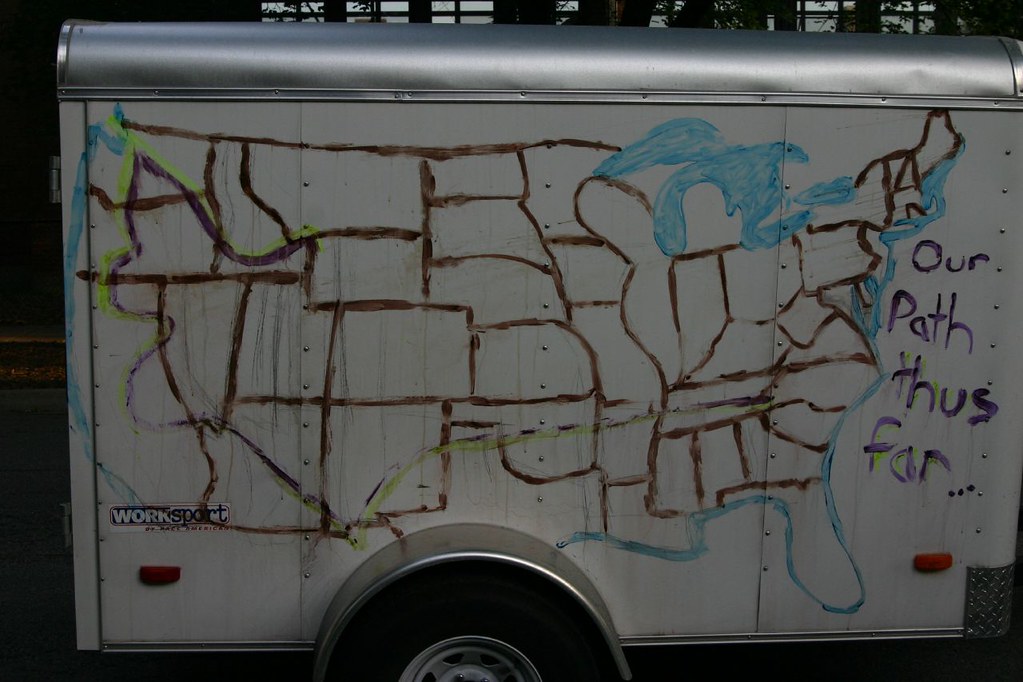The photograph captures the rear end of a small utility trailer, reminiscent of a U-Haul, though devoid of any such branding. The trailer's exterior is predominantly white with a metallic roof. The image appears to be dimly lit, adding a certain mystery to the scene. Visible is one of the trailer's wheels, accompanied by a modest logo on its left side that reads "Work Sport." 

The trailer's back features two reflectors and a notably large, crudely painted map of the United States. The map, largely colored in brown with splashes of blue outlining the coastlines and the Great Lakes, appears hastily crafted. Despite its rough appearance, the map details each of the U.S. states. Accompanying this artistic endeavor is text painted nearby that reads, "Our path thus far..." Additionally, streaks of green sporadically embellish the map, reinforcing the impression of a hurried, yet earnest, creative effort.